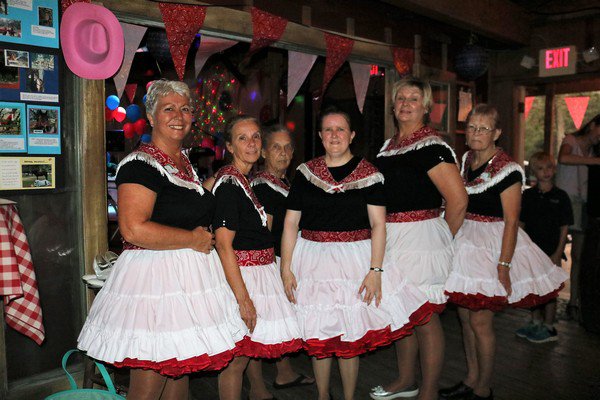In a cozy, celebratory restaurant setting, six older women are prominently positioned in the center of the image, all wearing matching uniforms. Their outfits consist of knee-length yellow skirts with a distinct red section at the bottom, red belts, black short-sleeved t-shirts, and red scarves with white edges draped elegantly around their necks. These women, standing close together, appear cheerful and unified, suggesting they may be part of a staff or performance group.

To the right of the image, a boy in a black t-shirt stands near the entrance, below an illuminated "Exit" sign. The backdrop includes a bulletin board adorned with photos and a hat hanging on the wall, adding character to the warm and inviting atmosphere of the restaurant. The image is awash with a palette of colors including light blue, pink, black, brown, red, white, purple, and light green, contributing to the lively and festive ambiance of the space.